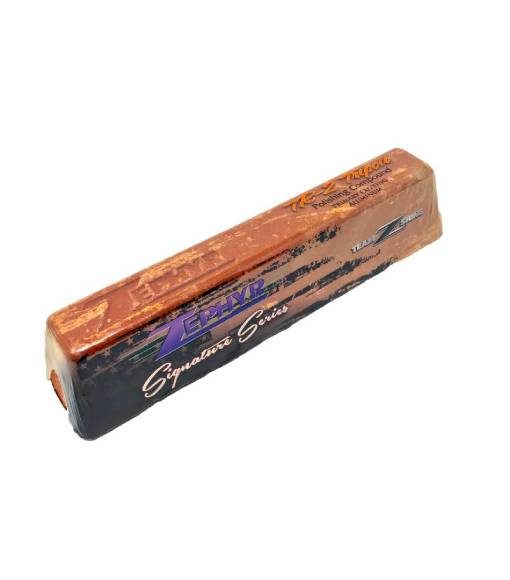The photograph depicts an oblong, brick-like object placed at an angle against a completely white background. The item, which is wrapped in clear plastic, has the appearance of a thinner gold bar or a block of cheese but is not food. The top of the object is rust-colored and features the text "Zephyr" in purple font, with "Signature Series" written below it in white font. The side of the object transitions from gray on one side to brown on the other and also displays "Zephyr" in purple. On the top right side, the text reads "Polishing Compound," indicating that this item is used for polishing purposes. Additionally, there is a mention of "Team Zephyr" on the right side of the item, and the visible end of the object forms a semicircle.